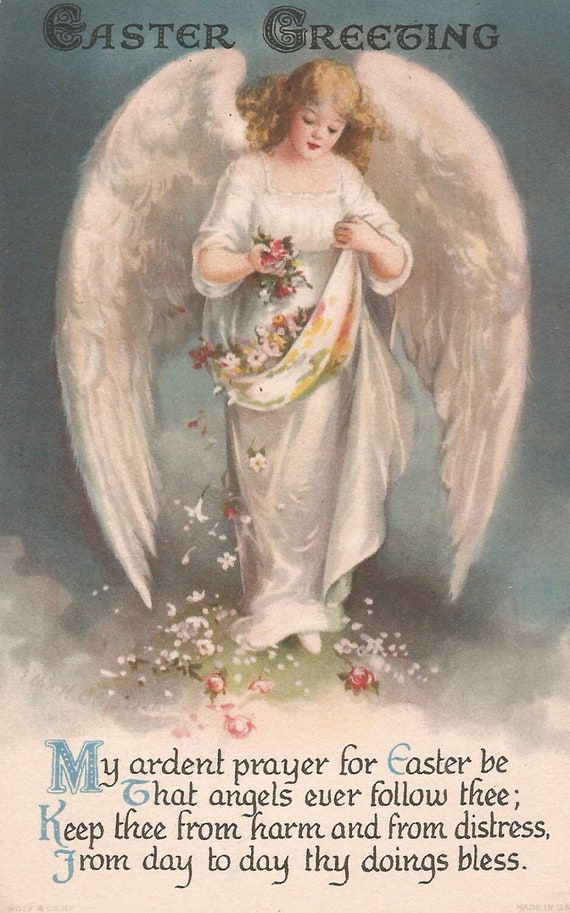The image depicts the front cover of an Easter greeting card, measuring approximately five inches high and three inches wide. It features a rich, detailed illustration set against a background of off-white and dark blue-gray clouds. At the top of the card, decorative typography spells out "Easter Greetings," with the capital letters E and G embellished with intricate spirals. 

Below this header, a feminine angel is depicted. She has long, curled blonde hair and light skin. Her large, white feathered wings gracefully arch above her head and around her sides. The angel is dressed in a flowing white gown and is holding pink flowers in her hands. She is also lifting part of her dress, which contains more flowers that are cascading to the ground. The ground beneath her is cloud-like, enhancing the ethereal quality of the scene.

At the bottom of the card, in a stylized text resembling old English or Celtic typography, a four-line verse reads: 
"My ardent prayer for Easter be 
That angels ever follow thee 
Keep thee from harm and from distress 
From day to day thy doings bless." 

This detailed imagery and poetic text combine to create a beautifully crafted Easter greeting card.